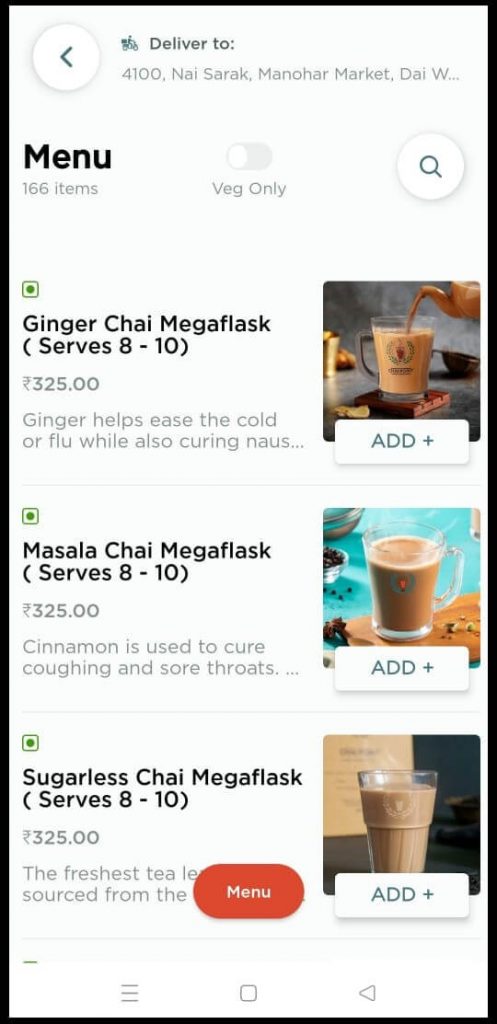This smartphone screenshot depicts a menu for chai offerings, prominently featuring three varieties of chai available in mega flasks that serve 8-10 people each. 

1. At the top of the screenshot is the delivery address written in a foreign language, alongside a search bar symbol opposite the word "menu."
   
2. The first item listed is a "Ginger Chai Mega Flask" priced at 325 units of the local currency. The accompanying image shows a person pouring ginger chai into a cup. The description highlights ginger's benefits in easing cold and flu symptoms as well as alleviating nausea.

3. The second item is a "Masala Chai Mega Flask," also serving 8-10 people. The image features a full cup of light-colored chai set against an aqua background, with the cup resting on a piece of wood. The description notes that masala chai contains cinnamon, which helps soothe coughing and sore throats.

4. The final listing is a "Sugarless Chai Mega Flask," similarly priced at 325 currency units and serving 8-10 people. The image shows a glass of chai on a black surface, with a piece of paper in the background. The partial description mentions the use of the freshest tea, sourced from an unspecified location due to the text being obscured by a tab labeled "menu."